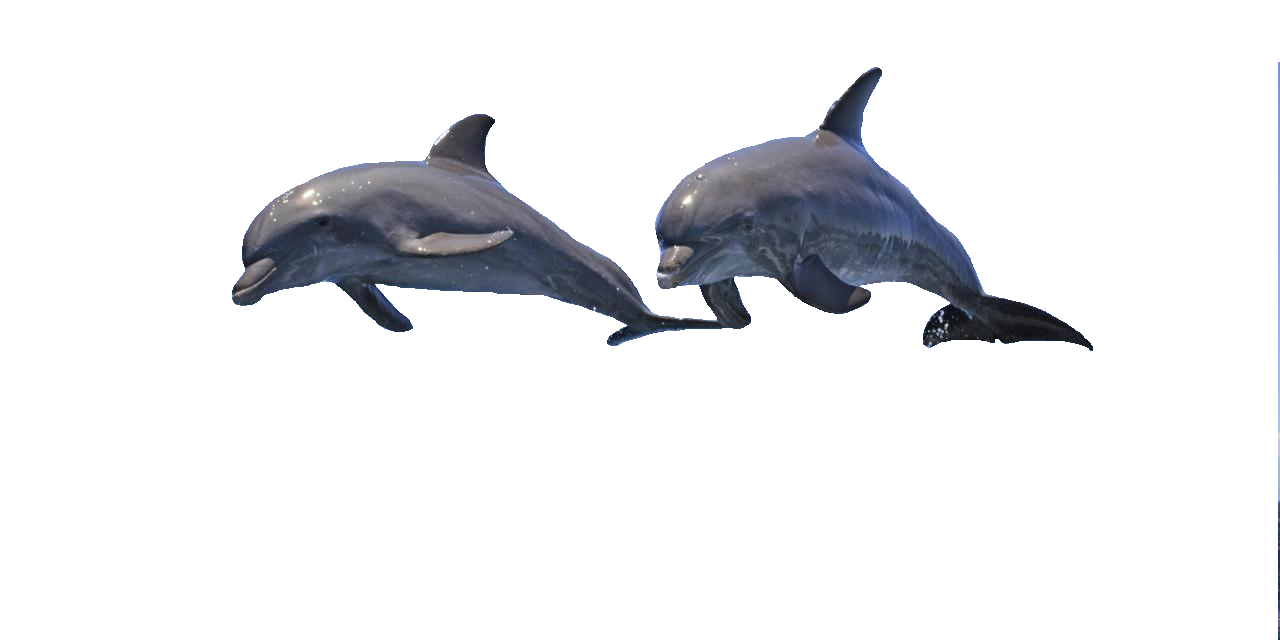The image features two dolphins, possibly bottlenose, presented against a perfectly white background, giving the impression that they have been removed from their natural water setting. The dolphins are nearly identical with magenta, purple, and grayish tones. They are shown mid-air, arched with their bodies angled towards the left. Each dolphin showcases a prominent dorsal fin, two side fins, and a robust tail fin. Notably, the eye of the left dolphin is visible while the right dolphin's eye is not. The image lacks a clear border except for a very thin strip of blue and black along the right edge. Despite some pixelation and roughness at the fins’ edges, the dolphins exhibit a dynamic presence, appearing as if they are gracefully floating or leaping side-by-side.